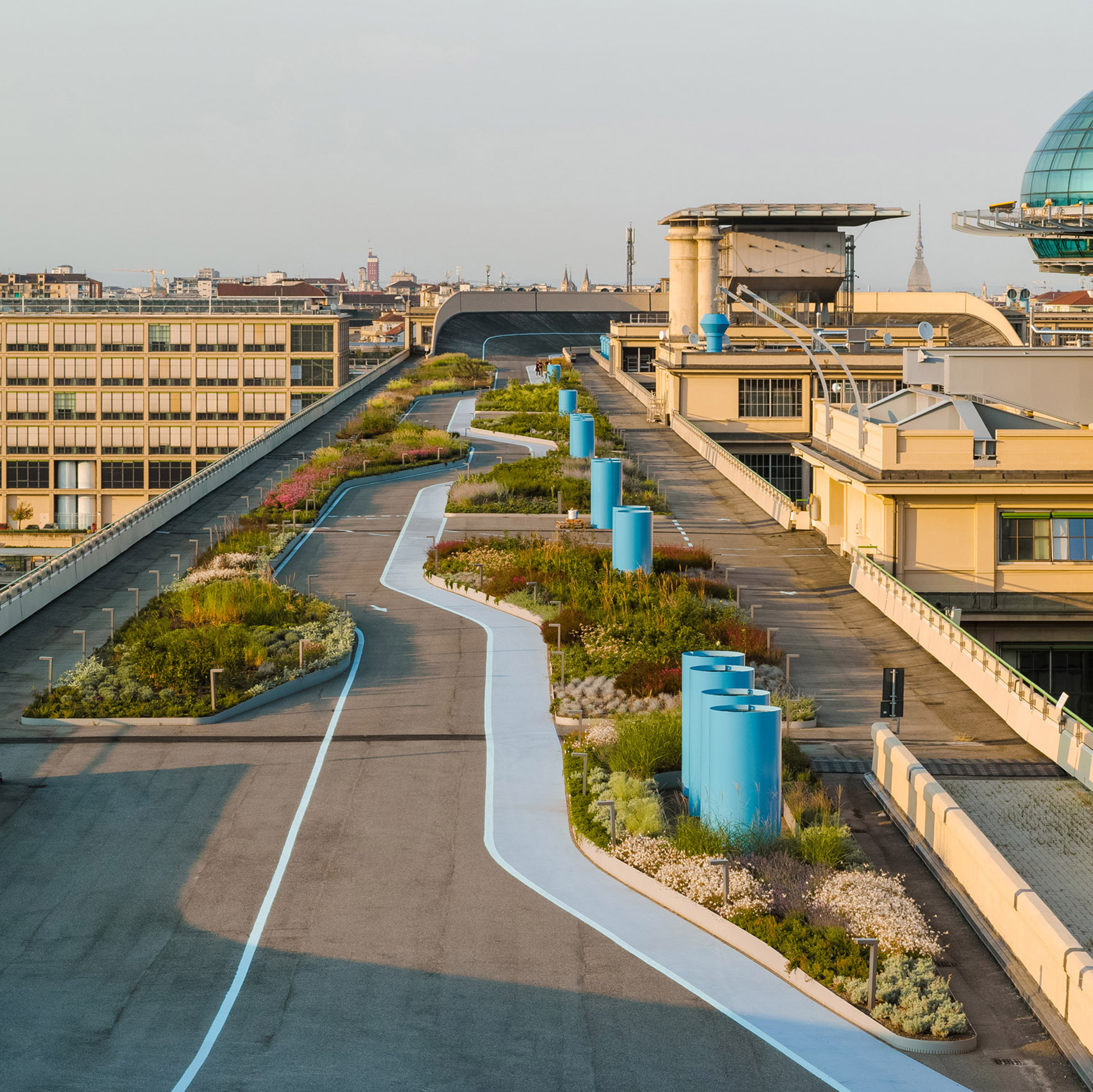The image depicts an elevated area that combines the characteristics of a rooftop garden and a pedestrian or bicycle-friendly bridge. The scene features well-maintained, structured gardens with curbs, filled with short white, light green, and red bushy flowers. These gardens are interspersed with at least 12 blue cylindrical objects arranged in a line from the front of the image to the back. The area surrounding these gardens is paved with black asphalt, marked with blue lines that resemble lanes and arrows suggesting directions. Notably, on the right-hand side, there’s a glimpse of a glass orb-like structure that could be an observation area. This setting seems to be part of an industrial area, potentially connected to an apartment or office building. The overall layout appears to prioritize pedestrian and bicycle traffic over cars, with pathways that likely descend to a road below.